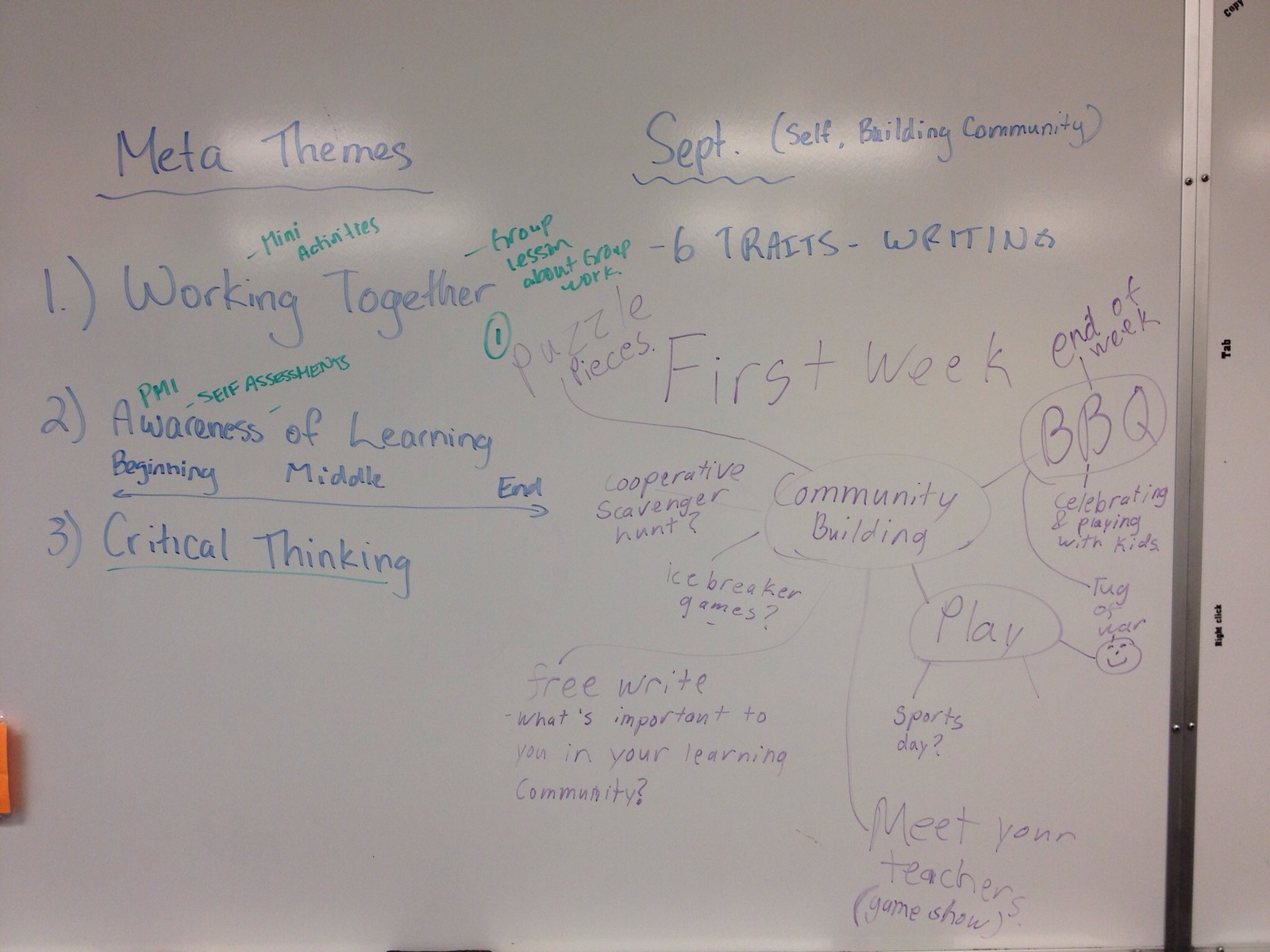In the photograph of a whiteboard, handwritten in various colors, multiple detailed items highlight a learning and community-building plan. At the top left, the title "Meta Themes" is emphasized in blue lettering, followed by three key points: 1. Working Together, 2. Awareness of Learning, and 3. Critical Thinking—all underlined for importance. Below "Awareness of Learning," arrows point to the words "beginning," "middle," and "end," indicating a progression or cycle.

On the right side of the whiteboard, also in blue, the heading "September" leads into a list that includes "Building Community" and "Six Traits Writing." In purple, a word cloud or bubble plot radiates from the central term "Community Building," branching into various activities such as "Barbecue" on the right, "Play" and a circled smiley face with "Tug of War" above it at the bottom, "Cooperative Scavenger Hunt" to the left, and "Ice Breaker Games" at the bottom left. Additionally, "Meet Your Teachers" with a note "like game show" extends from "Community Building." There's a note denoting ideas for activities in the first week. Scattered on the left, there are unreadable notes in green, adding to the brainstorming nature of this detailed and comprehensive plan for fostering community and enhancing learning.